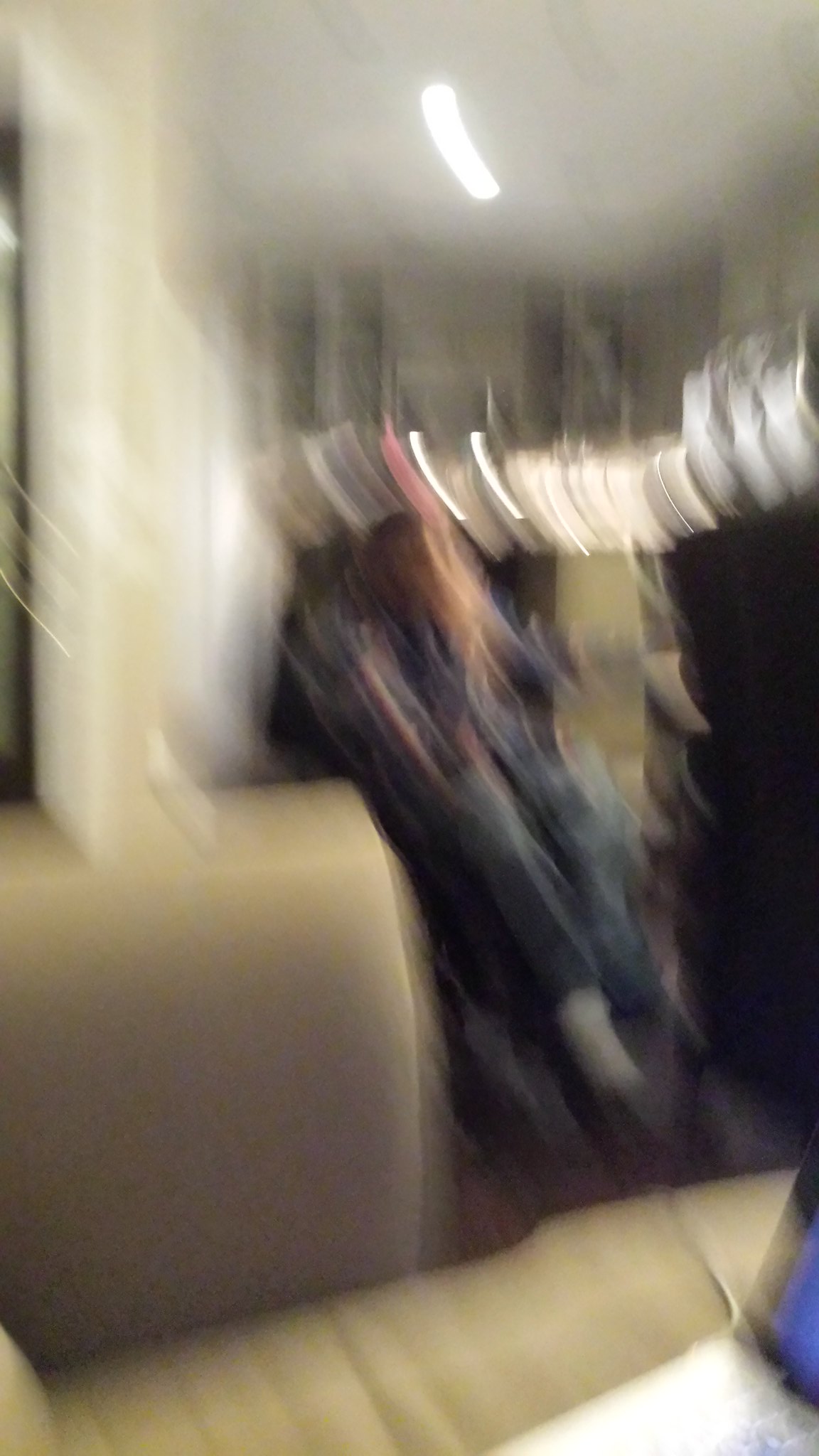The image captures a scene in motion, characterized by a distinct motion blur that drags elements downward and slightly to the right. In the foreground, there's a tan leather couch, its contours softened by the blur. In the middle ground, a person with long tan-brown hair is faintly visible. They appear to be dressed in a blue top, blue jeans, and white socks, possibly seated in a black chair. The background features tall windows, hinting at a spacious and well-lit environment. The overall effect gives the impression of a dynamic moment, frozen in a rush of motion and color.